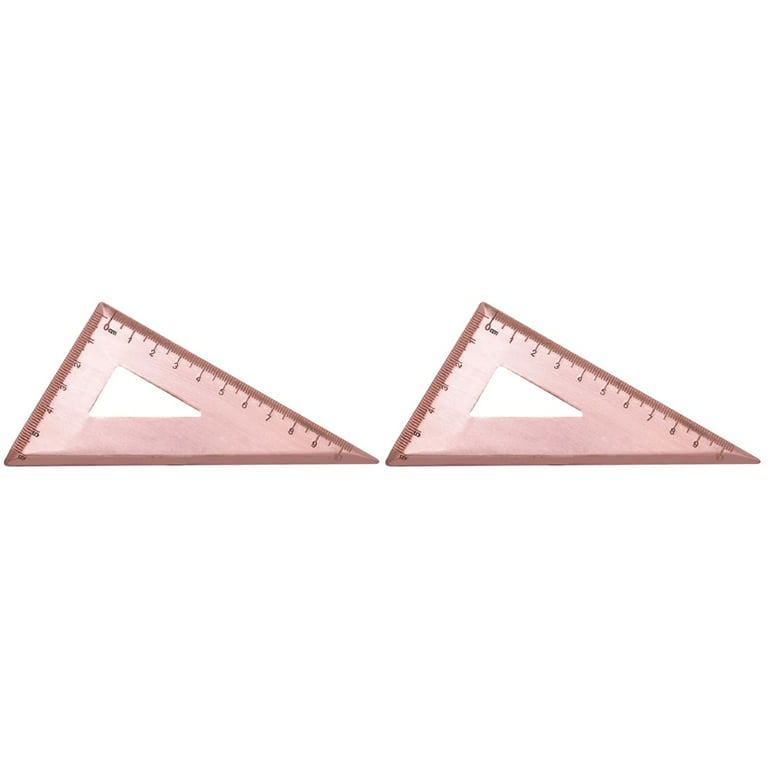The photograph showcases a pair of right-angle, 60-degree set square geometry instruments positioned side by side against an entirely white background. Both instruments are made of a transparent pink or amber plastic and measure approximately 10 inches on the long side and 6 inches on the shorter side. Each has numbers marked on the sides that form the right angle, ranging from 0 to 10 inches on one side and 0 to 6 inches on the other. Notably, each square has a cut-out middle section in the same shape as the instrument itself, which serves as a convenient grip for handling. Their positioning resembles the arrangement of the top left corner of a pizza slice laid down flat.